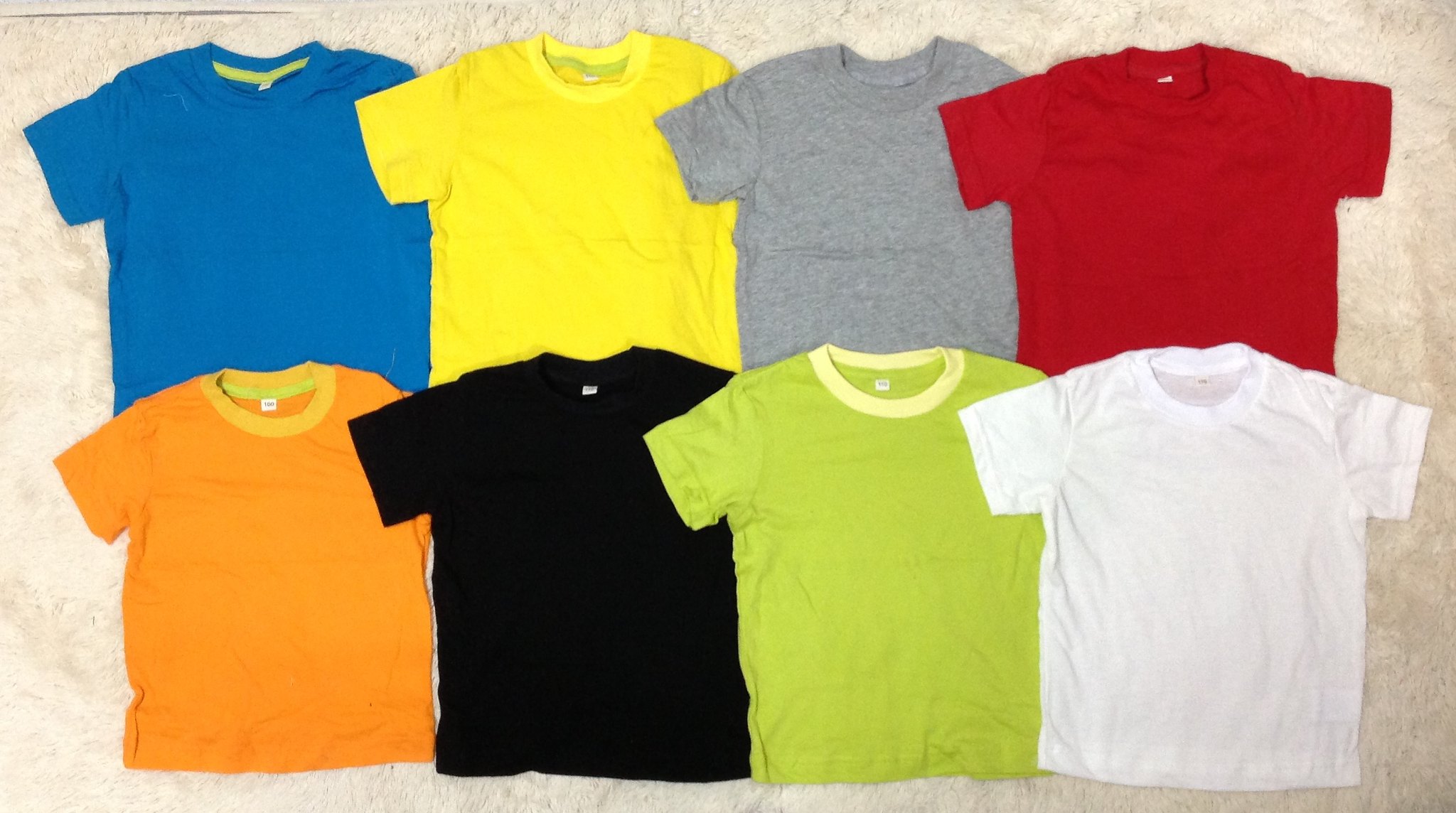This is a horizontal photograph of eight boxy short-sleeve t-shirts laid out neatly on a cream-colored, textured background that resembles a lightly off-white or fluffy surface. The t-shirts are arranged in two overlapping rows. The top row, from left to right, features a medium blue t-shirt with a yellow internal collar, a bright yellow t-shirt, a gray t-shirt, and a red t-shirt. The bottom row, continues from left to right with an orange t-shirt, a black t-shirt, a bright green t-shirt with a lighter green collar, and a plain white t-shirt. Each t-shirt is fully stretched out, allowing the circular necks and short sleeves to be clearly visible. The angle of the photograph is from above, capturing the t-shirts laid on a flat surface, slightly wrinkled and overlapping each other at the sleeves.